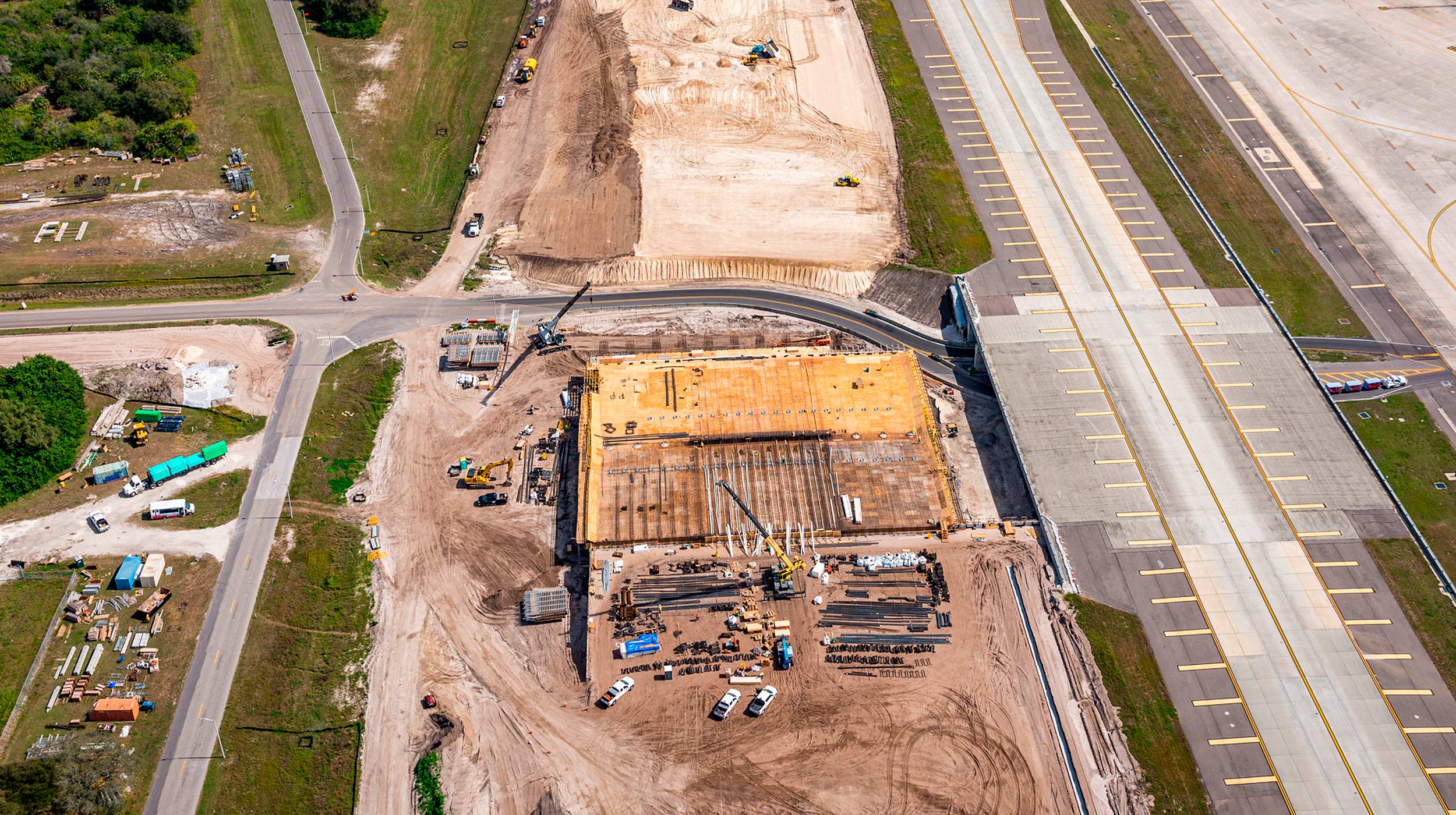The image depicts an aerial view of a construction site adjacent to an airport. Centered in the photograph, a U-shaped building is under construction, visible with raw wood elements and surrounded by organized piles of building supplies on a cleared, dirt expanse. Numerous construction and support vehicles, including a crane, are actively involved in the site, indicating significant ongoing development. To the left of the construction area, an airport taxiway and ramp are evident, with a distinctive taxiway bridge crossing over a road that runs underneath. On the right side of the image, a long concrete road adorned with horizontal and vertical yellow stripes curves into the distance, flanked by rows of parking spaces. Surrounding the entire construction zone is a mix of green and brownish-green grass, adding a natural border to the industrial scene. The high contrast between the bustling construction site and the structured airport elements provides a detailed snapshot of coordinated urban development.